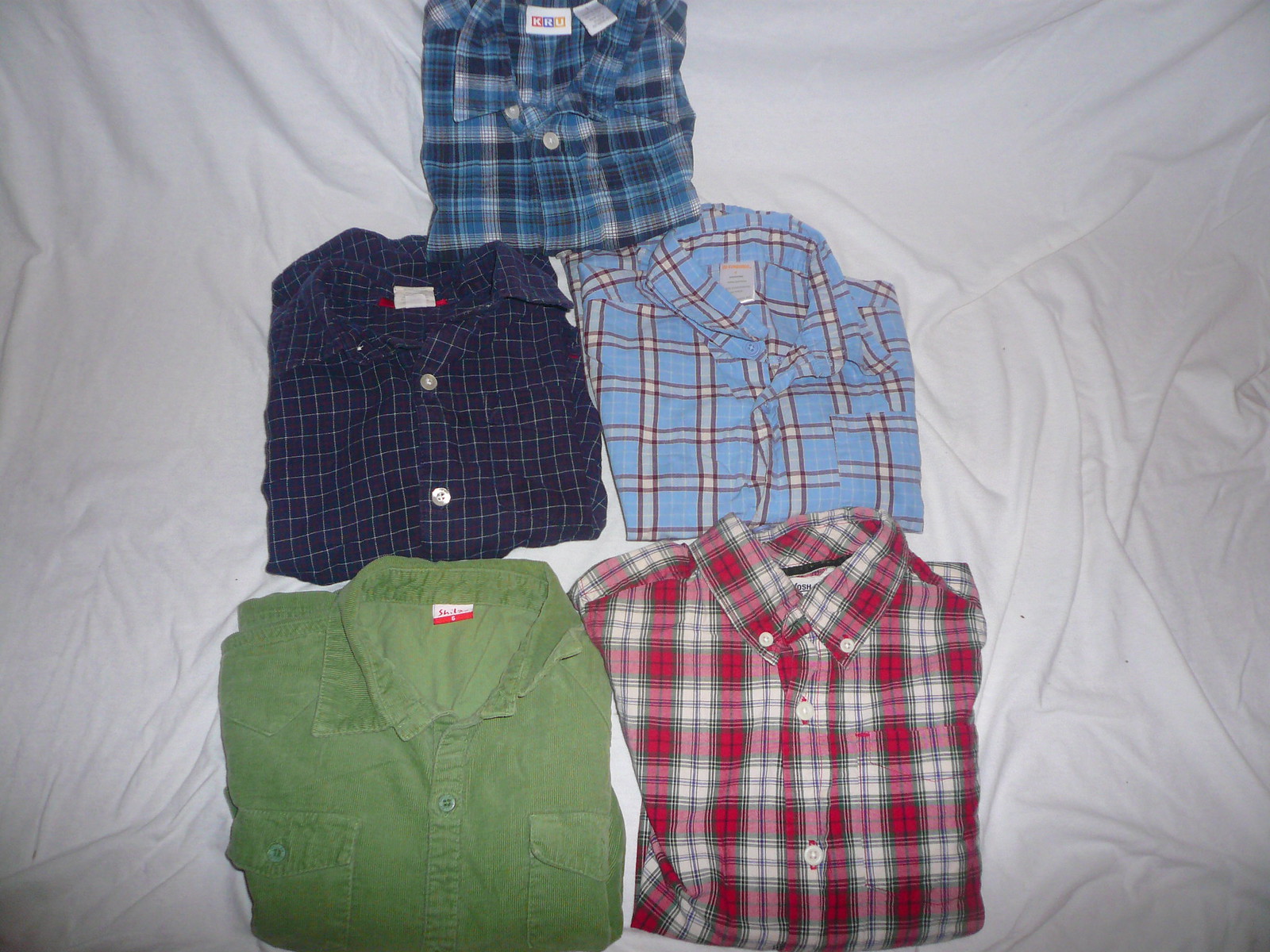The image is a color photograph taken from above, depicting five children's button-down collared shirts, all folded and displayed on a wrinkled white sheet, likely the bottom sheet of a bed. The shirts are arranged in two rows of two, with a fifth shirt at the top. The top shirt features a blue, gray, and navy check pattern with a "KRU" tag. In the second row, the left shirt is dark blue with a white check, while the right shirt is light blue with a windowpane check, tagged "Gymboree." In the bottom row, the left shirt is a solid medium green with patch pockets, while the right shirt is a red and white plaid shirt with a button-down collar. The shirts are unevenly folded, with visible folds and creases, mirroring the rumpled surface of the sheet they rest upon.